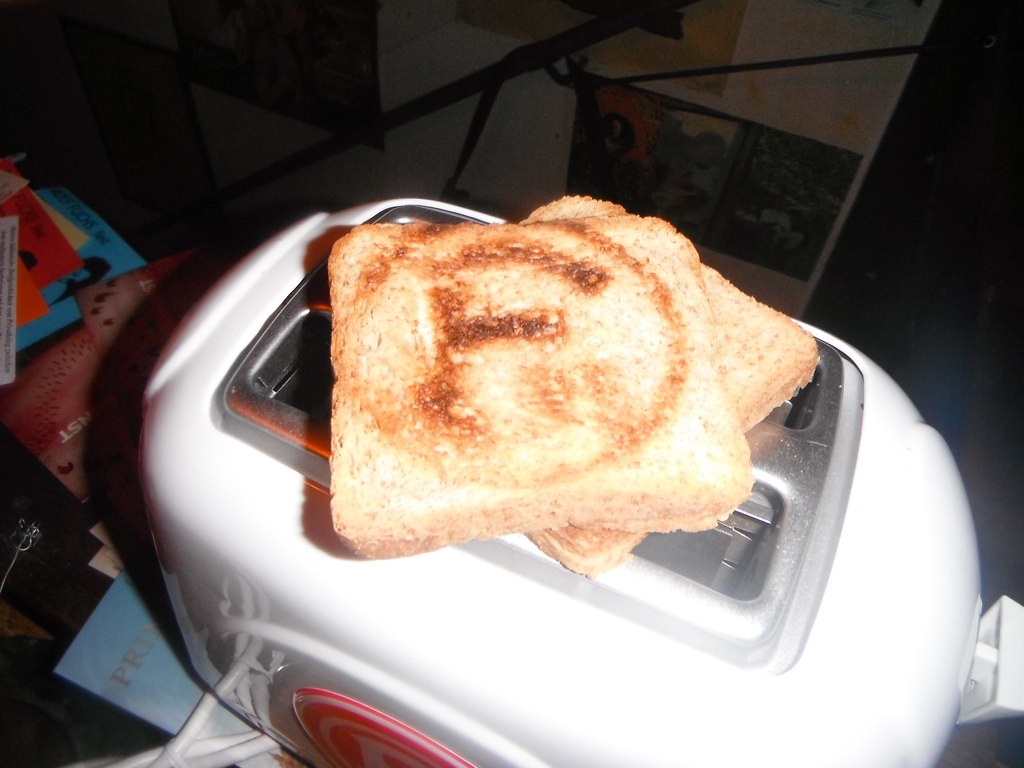This detailed landscape-format photograph, visually cluttered and slightly overexposed due to flash, captures a white toaster with a hint of pink on its sides, partially obscured by the framing of the shot. On top of the toaster, slightly ajar from each other, rest two pieces of toasted white bread. These pieces feature a distinct pattern: a burnt, brown circle encompassing a letter "F," suggestive of a brand emblem that is faintly visible on the toaster's left side. Surrounding the appliance is an assortment of colorful, indiscriminate brochures and advertisements, adding to the general messiness of the environment. The image, taken from an overhead diagonal angle, prominently focuses on the uniquely marked toast while providing a glimpse into the chaotic countertop filled with various papers.